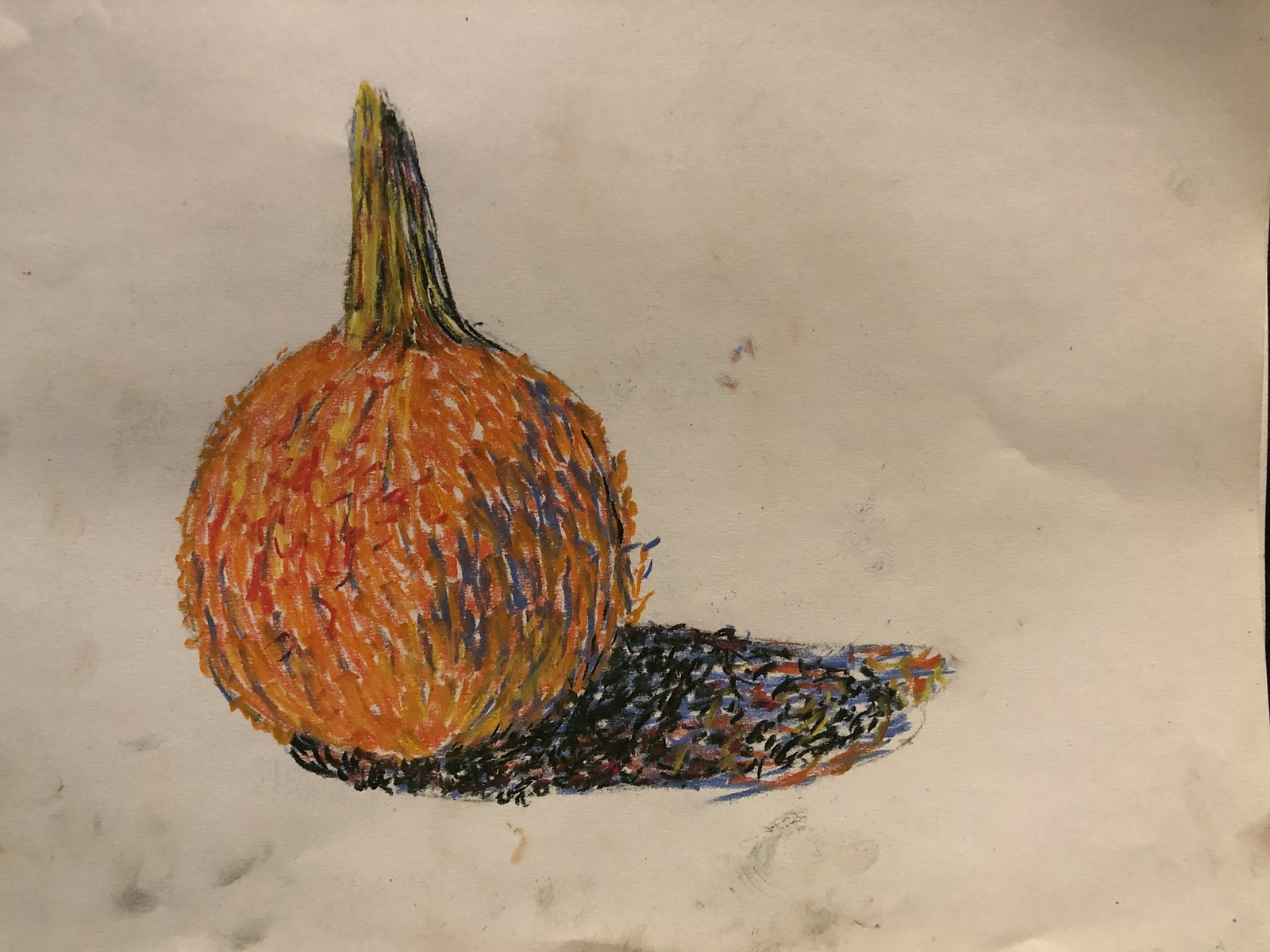A detailed drawing depicts a rich orange root vegetable, possibly a gourd, with a thick, textured stem that is characteristic of many root vegetables. The vibrant orange hue of the vegetable contrasts beautifully with the dark shadow beneath it, suggesting depth and dimension. The artwork, rendered in wax crayon and possibly accented with markers or pens, exudes a rich textural quality, especially noticeable in the stem. Various shades and small bits of color are skillfully blended throughout the image to enhance its realism. The vegetable appears untouched, ripe, and in excellent condition, capturing the artist's meticulous attention to detail.